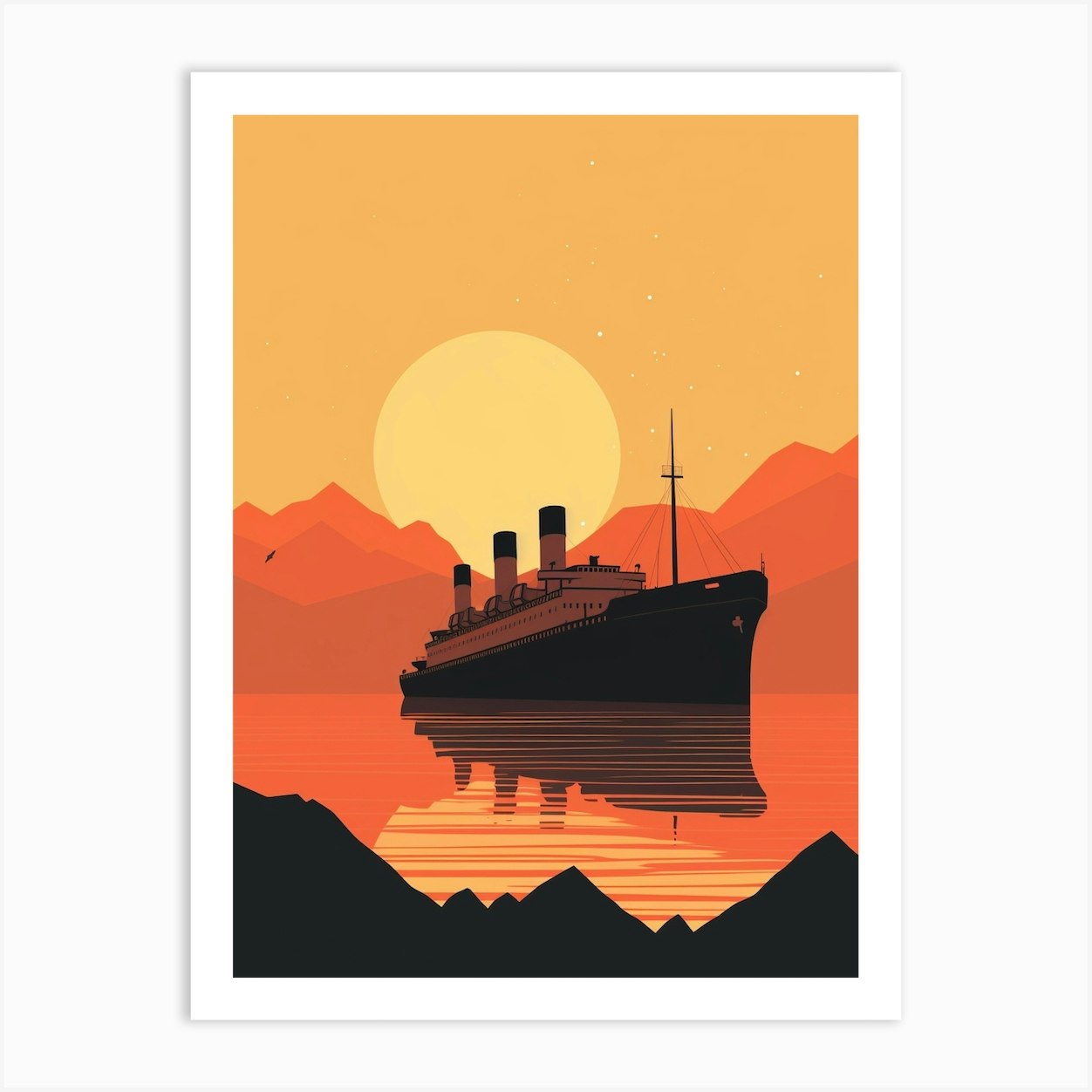This detailed painting depicts a large ship at sea, rendered in vibrant yellows, oranges, and blacks. The ship, prominently featured in the center, is black with a white top and three large white smokestacks extending from its deck. Set against an isometric perspective, the ship’s reflection can be seen in the orange and yellow waters below, characterized by distinct black reflections. Behind the ship, an orange and brown mountain range stretches across the horizon, silhouetted against a yellow sky dotted with white stars. A large yellow sun is beginning to set behind this mountainous backdrop. In the foreground, the painting includes black hills and additional mountain peaks, adding depth to the composition. The entire scene is framed by a thin white border, enhancing its crisp, illustrative quality.